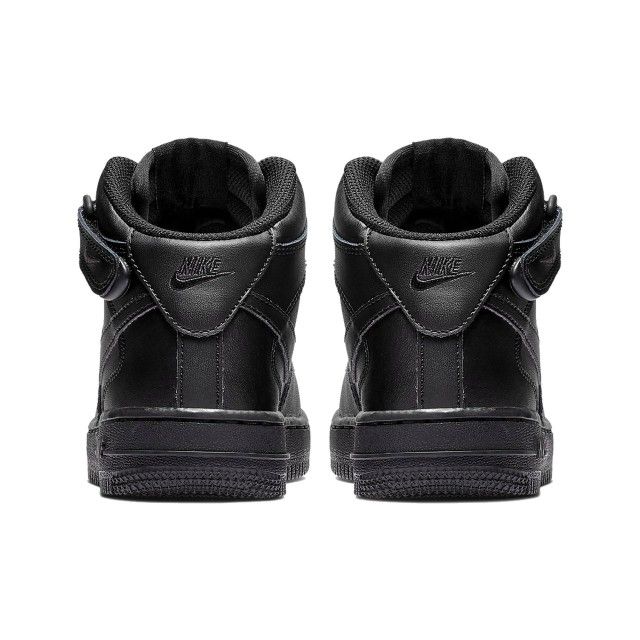The image features a pair of high-top black Nike sneakers displayed against a white background. These shoes, likely designed for running or other athletic activities, are crafted from black leather with black stitching. The insides feature black fabric cushioning for added comfort, and the tongue and ankle portions are lined with black mesh. Each shoe has a secure Velcro strap adorned with a Nike logo, resembling a check mark. The soles are black, probably made of rubber, and have a fine tread pattern composed of X's or K's. The backs of the sneakers prominently display the Nike logo, impressed into the leather, adding to the overall sleek, monochromatic design.